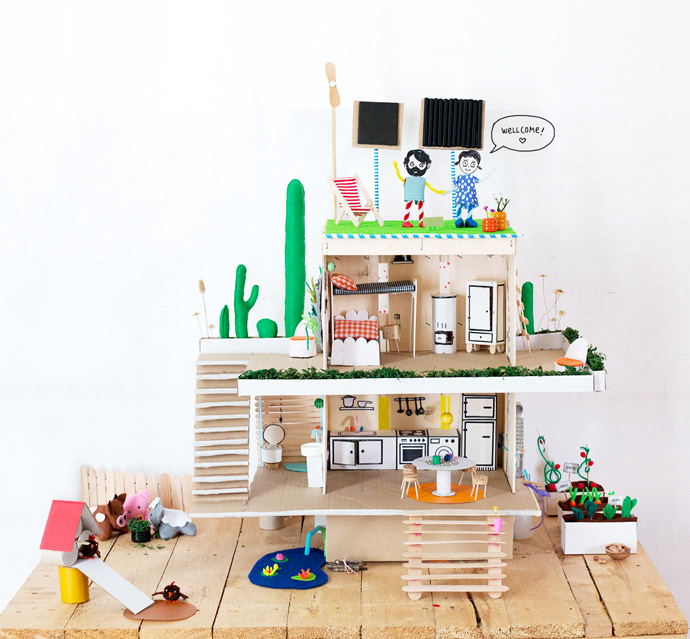The image is a detailed photograph of a whimsical, multi-level dollhouse with each floor and outdoor area adorned with playful details. The dollhouse stands on a surface made of rough, unvarnished wooden boards arranged vertically, simulating a yard with elements such as a chicken coop, cows, pigs gathered around a bucket, and a small pond.

The dollhouse appears to have three levels. The bottom level serves as a kitchen and dining area with a small white table and chairs, outlined drawings of a sink, stove, and refrigerator, and a bathroom to the left. A tan ladder is positioned at the front, connecting the different levels.

The second level features a uniquely designed bedroom with beds arranged perpendicularly. The top bunk is oriented horizontally while the bottom bunk runs vertically. Adjacent to the beds is a dresser and a small table, with a patio area to the right adorned with a white chair with an orange cushion. Green cactuses flank both the left and right sides of this floor.

On the top floor, there is an outdoor patio covered with green astroturf, equipped with a chair, two tall monitors, and cardboard cut-outs of a man and a woman beneath the monitors. The man, positioned on the left, has black hair, a black beard, and wears a blue shirt. The woman on the right has curly black hair, wears a blue dress with white polka dots, and blue shoes. Both figures sport exaggerated features with big googly eyes and seem to have limbs made of colorful candies like Twizzlers and yellow spaghetti for arms. The woman holds a speech bubble saying "welcome," adding to the playful and welcoming aesthetic of the dollhouse.